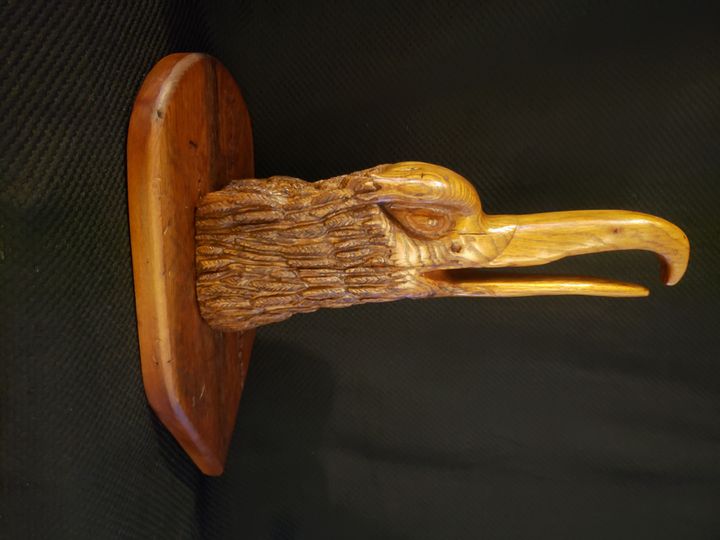This image depicts a detailed carved wooden sculpture of an eagle's head mounted on a small wooden base, ideal for wall display. The eagle's head, which is prominently shown in a side profile, features meticulous carvings that highlight the intricate details of its long, curved beak, piercing eye, and textured feathers along the neck. The sculpture is predominantly brown, with the beak and facial features rendered in a lighter yellowish-brown hue, while the darker brown details emphasize the eyes and feathered texture. The base suggests it might function as a decorative piece or coat hook, though its exact purpose remains ambiguous. The background is black, further accentuating the craftsmanship and aged appearance of the wooden plaque, which hints at mid-20th-century origins.